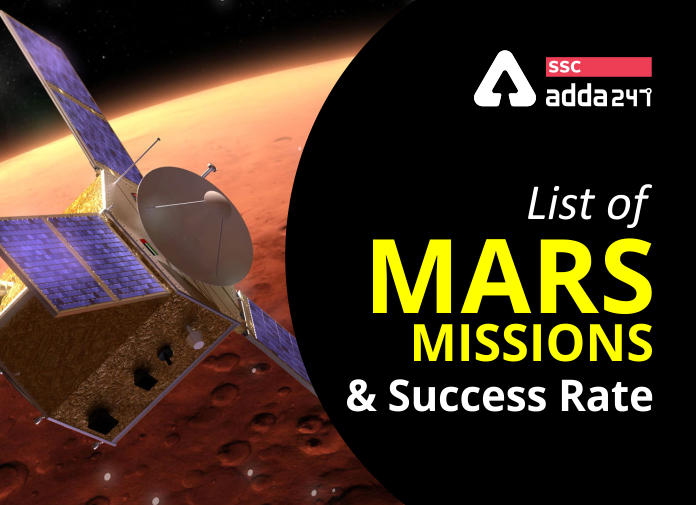The image is a detailed infographic, likely designed for a YouTube video or a PowerPoint presentation lecture series, showcasing a CGI depiction of a Mars mission. On the left side, a prominent, close-up view of the red, cratered surface of Mars dominates the frame, emphasizing its distinctive orange-red hue. Floating above Mars is a gold-colored, hexagonal-bodied satellite featuring three blue, reflective solar panels and a white satellite dish. The right side of the frame transitions to a solid black background where white and yellow text reads "List of Mars Missions and Success Rate." At the top right, within a rounded triangle icon with a red bar, there's the text "SSC ADDA 247," providing context for the visual as part of an informational series or event. The design is cleanly divided by a subtle circular curvature, enhancing the separation between the image of Mars and the satellite on the left, and the descriptive text on the right.